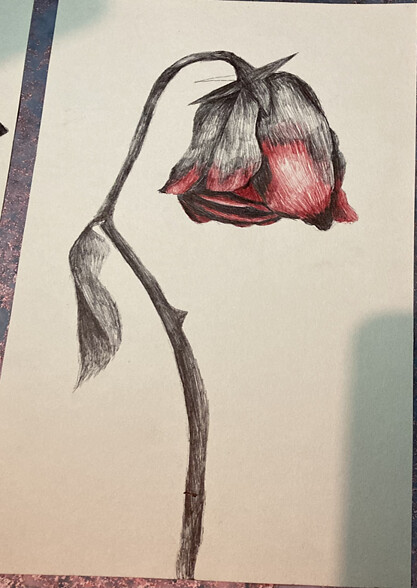The photograph captures a detailed pencil sketch of a withered rose on an off-white rectangular sheet of paper. Dominating the image, the thorny stem originates from the bottom, curving up and forming a J-shape, before a dramatic downturn. The stem, shaded intensely in black and gray, accentuates the lifeless nature of the plant. A single leaf, equally shadowed in black, droops morosely from the left side of the stem. At the top, the bloom hangs despondently, with its petals transitioning from dark, heavy sketch marks to delicate hints of red and white at their tips, adding a touch of ethereal beauty to the decaying flower. A shadow, likely cast by the device taking the photograph, falls across the bottom right corner, tinged with a faint light green hue, introducing an element of depth and realism to the composition.